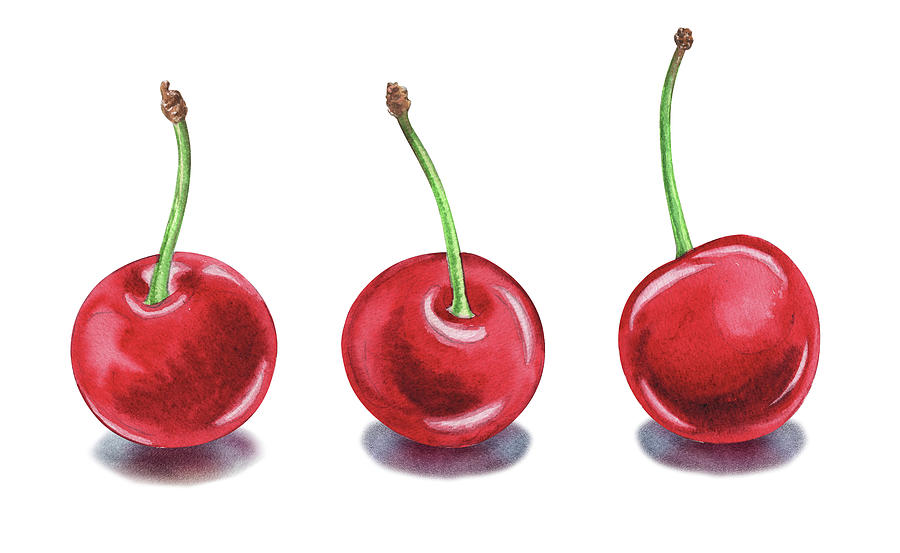This is a detailed illustration of three vibrant, red cherries, positioned in a neat row. Each cherry is depicted with its stem still intact, arching gracefully upward. They are arranged upright on a flat surface, creating a natural alignment. A subtle shadow beneath each cherry suggests depth and adds a touch of realism to the illustration. Two of the cherries are oriented forward, clearly showcasing the small, concave area where their stems connect to the fruit. The third cherry, positioned on the right, is turned slightly away from the viewer, concealing its stem indentation and adding a dynamic element to the arrangement.